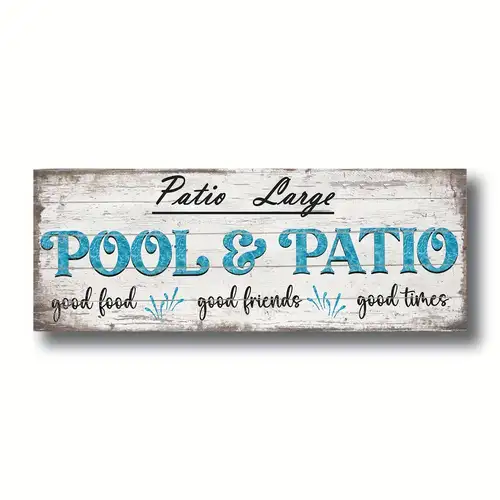The image features a rustic, aged white wooden sign with patches of gray, giving it a weathered appearance. The sign's dimensions are approximately three feet wide by one foot tall. At the top, in black cursive script with an underline, it reads "Patio Large" with the 'P' and 'L' capitalized. Below this, in all-capital blue text, it reads "POOL AND PATIO" with decorative elements on the letters 'O' and 'P'. The third line, also in black cursive, states "Good Food, Good Friends, Good Times," with blue splashes of water separating these phrases. The sign is centrally positioned against a white background.